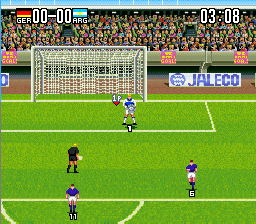The screenshot is from an early 90s Super Nintendo soccer video game, featuring a match between Germany and Argentina. The game clock shows 3:08 with the score tied at 0-0. The scene captures the goalkeeper in a white and blue uniform about to kick off, while two players in blue jerseys and another in a black shirt are positioned nearby. The vibrant green field is enclosed by silver or gray concrete barriers, crowded with spectators. Behind the goal, a single banner reading "Jaleco" in blue on white is visible. At the top of the screen, the scoreboard highlights the teams' flags, indicating the countries, and the time. Red signs with white text are also present on the perimeter walls.